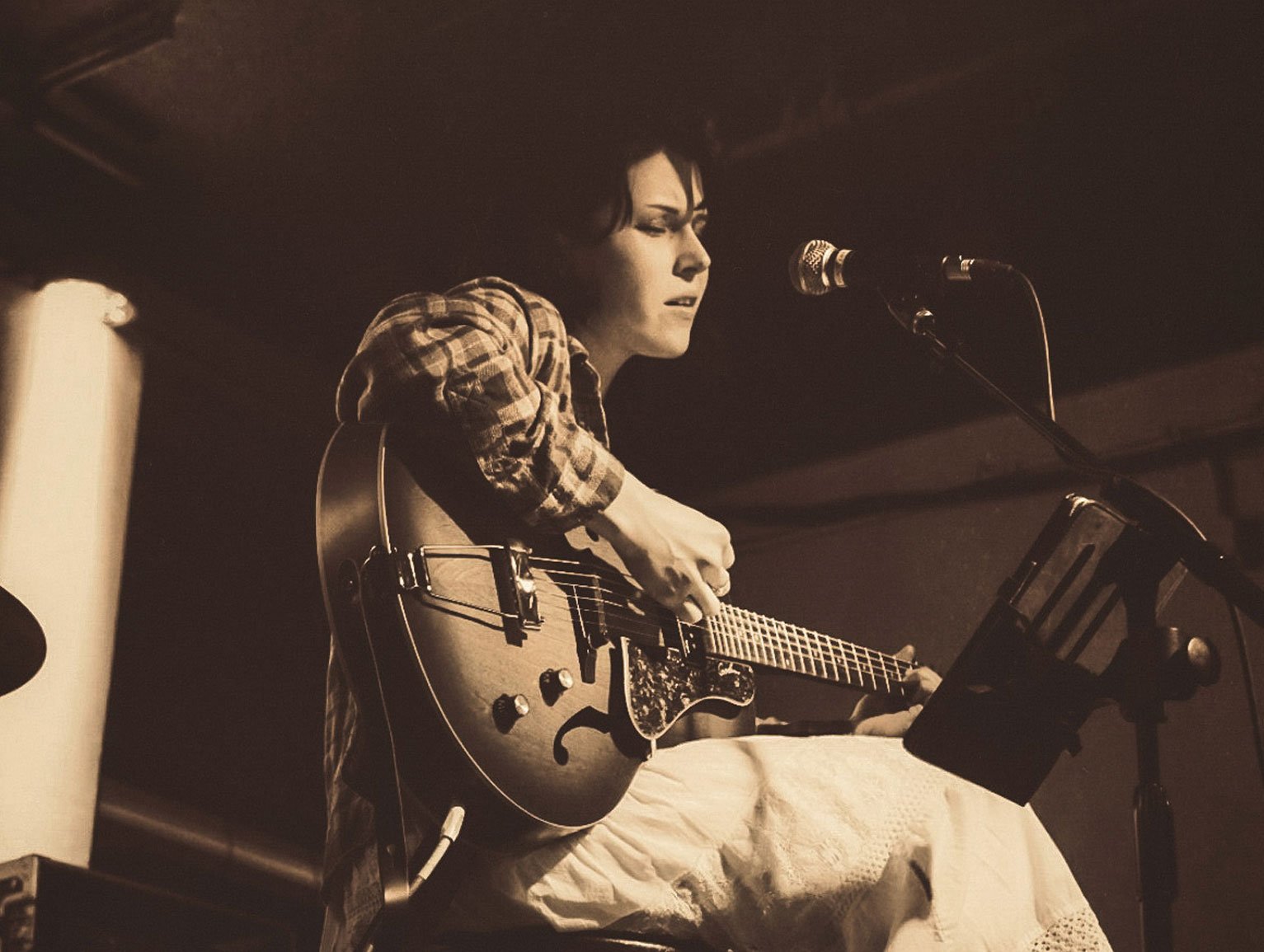In this sepia-toned photograph, a white woman with short black hair is captured in a moment of musical focus. Seated from a side view in a dimly lit setting, likely a music studio or stage, she strums an electric-acoustic guitar while singing into a microphone placed in front of her. Her eyes are closed, adding an element of deep concentration as she glances down at a music stand holding notes or lyrics. She is dressed in a plaid long-sleeve shirt and a loose, lacy white skirt. The guitar is connected to an amplifier, indicating a blend of acoustic and electric elements. The intimate atmosphere and detailed expression suggest a soulful, possibly country, performance.